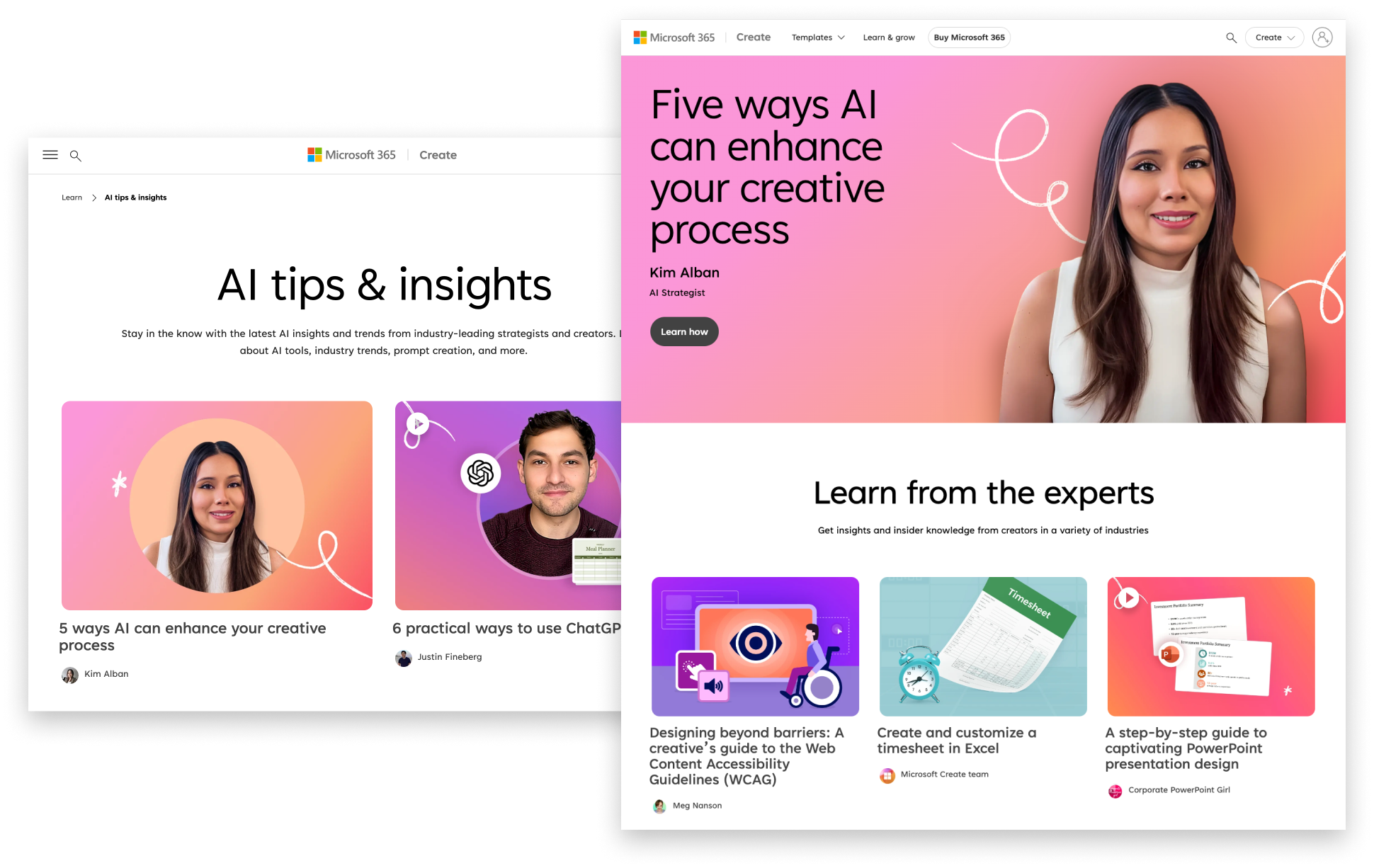The image displays two screenshots from websites under the Microsoft 365 banner, both prominently featuring the recognizable orange, green, blue, and yellow Windows logo.

The left screenshot is titled "AI Tips and Insights," inviting users to stay updated with the latest AI trends and insights from industry-leading strategists and creators. It outlines topics such as AI tools, industry trends, and prompt creation. Additionally, it showcases two articles by different creators: "Five Ways AI Can Enhance Your Creative Process" and "Six Practical Ways to Use ChatGPT."

The right screenshot highlights an article titled "Five Ways AI Can Enhance Your Creative Process," written by AI strategist Kim Alban. It features a gray "Learn How" button, encouraging users to gain insights and insider knowledge from experts across various industries. Suggested articles include "Deciding Beyond Barriers: A Creative's Guide to the Web Content Accessibility Guidelines,” "Create and Customize a Timesheet in Excel," and "A Step-by-Step Guide to Captivating PowerPoint Presentation Design."

The background of both images is predominantly white, with black text and vibrant purple and pink designs adding a colorful backdrop to the displayed articles.